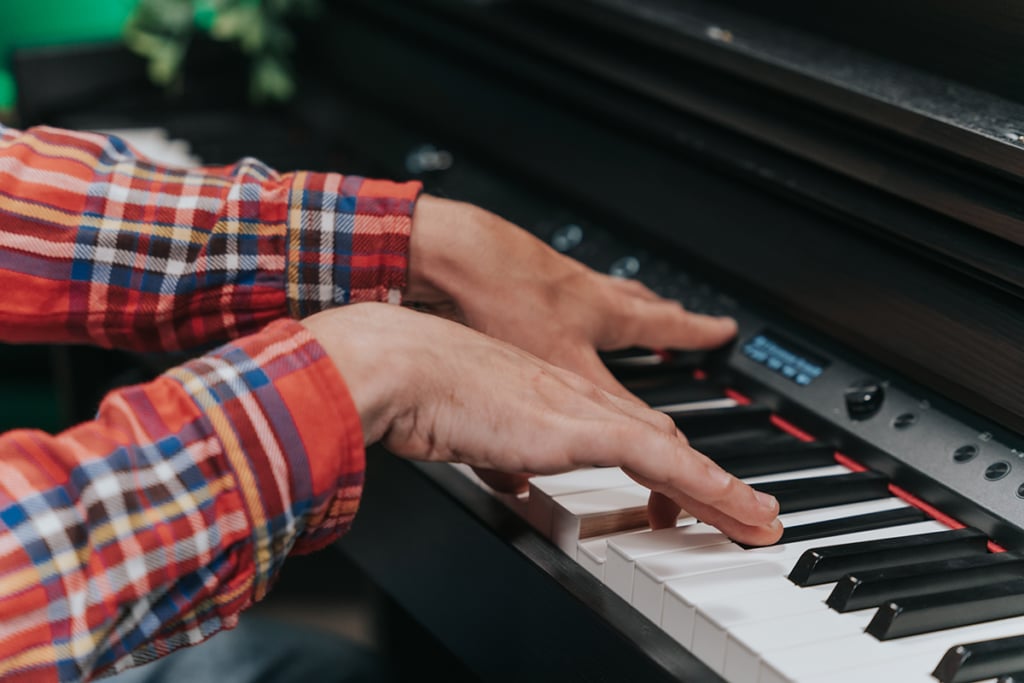In this detailed and intimate image, we see the close-up hands of a keyboardist actively playing an electric keyboard. The hands, which appear to be those of a white man, are poised over the familiar white and black keys. The keyboardist is wearing a striking long-sleeved flannel shirt, predominantly red, adorned with a pattern of blue, white, black, and yellow intersecting stripes forming checked boxes. The shirt’s cuffs extend to the wrists, highlighting the detailed plaid design. Only a glimpse of the person’s gray pants is visible beneath the keyboard. The keyboard itself is a digital model, featuring an LED display, numerous knobs, and buttons above the keys, providing a stark juxtaposition to traditional pianos. A distinctive red line marks the top of the keys. In the background to the upper left, a green wall and possibly a potted plant or green leaves subtly emerge into the frame, adding a touch of natural texture to the scene. The overall composition focuses on the act of playing, blending vibrant textiles and digital instrumental elements.